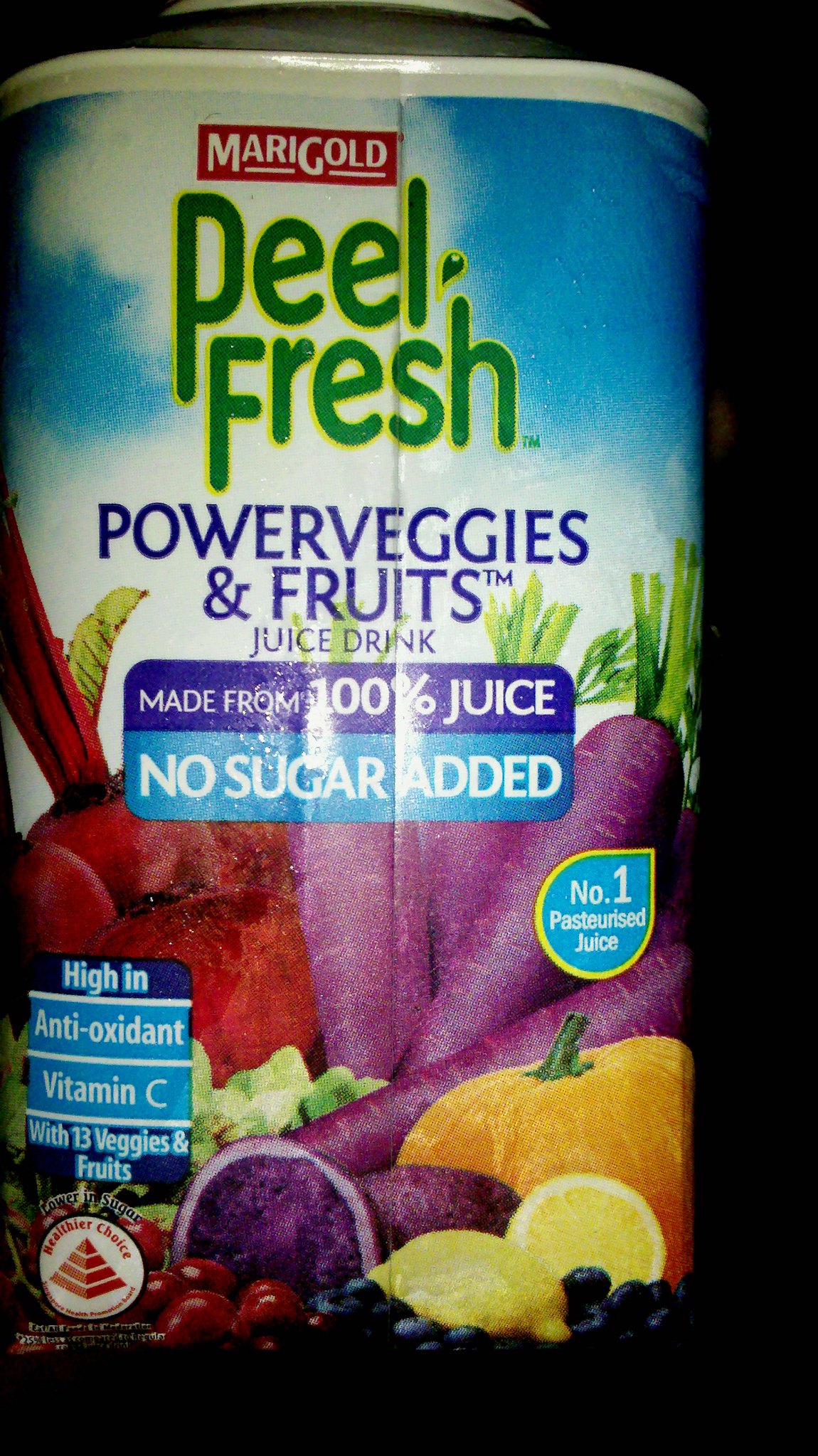This is a photograph of a rectangular juice label. The bottom and right sides of the photograph are shrouded in black, framing the label which occupies the rest of the image. At the top of the label, there is a white strip, followed by an illustration of a blue sky adorned with white, puffy clouds. Centered below the top in a bold red rectangle with white lettering, it reads "Marigold." Beneath this, in green text, it says "Peel," followed by the word "Fresh" in a larger font. Further down in purple text, it reads "Power Veggies," accompanied by "In Fruits" underneath it. The phrase "Juice Drink" is prominently displayed below that.

There is a wide horizontal rectangle in the middle of the label. The top half of this rectangle is purple with white text that declares "Made From 100% Juice." The bottom half has a blue background with the words "No Sugar Added" in white text.

The lower section of the label is dominated by a vibrant illustration of assorted fruits and vegetables. On the right-hand side, with their leafy tops visible, are purple carrots. Just beneath them lies an orange pumpkin. Spanning the bottom portion of the label, there are blueberries and cherries interspersed throughout, alongside a whole lemon and a halved lemon positioned slightly behind it. Additional vegetables such as a red vegetable on the left and some green lettuce in the middle further enrich the array of produce depicted in this lively, colorful composition.